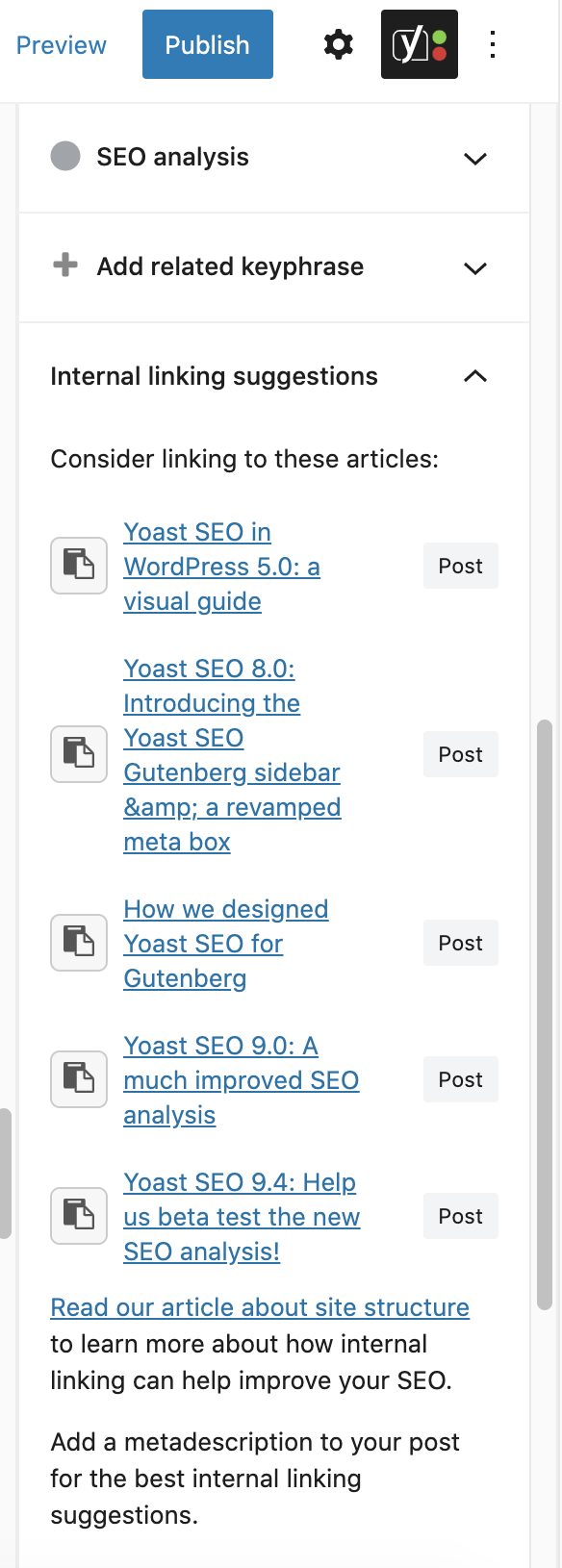**Image Caption:**

The image showcases a webpage interface with various functional elements detailed below:

- In the upper left-hand corner, there's the word "Preview" displayed in blue font.
- Adjacent to the "Preview" text, on the same navigation bar, is a "Publish" button in blue with white font.
- Following this, there is a gear icon separated by some space.
- Next to the gear icon, there's a black box. Within the black box, a white box is centrally located, featuring a blue "Y" in its middle.

Below this navigation bar, a series of sections is presented:

1. **SEO Analysis:** This section has a drop-down arrow indicating additional options or details can be revealed.
2. **Add Related Key Phrase:** This section includes a plus sign to the left of the text and a drop-down bar for further interaction.
3. **Internal Linking Suggestions:** This section is currently expanded. At the top of the expanded view, the text indicates recommendations for linking to specific articles. 

The list of articles suggested for internal linking includes five items, each with a clickable hybrid link to navigate to the respective article. To the right of each article link is a "Post" button for further actions.